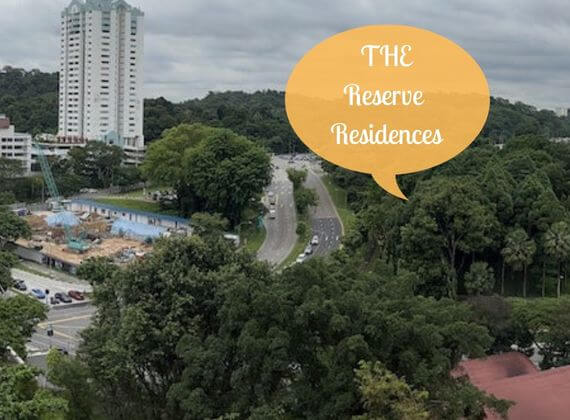The image captures an overview of "The Reserve Residences," featuring a mix of natural and urban elements. In the lower right corner, a red rooftop peeks into the frame, likely belonging to single-story buildings that resemble a motel, with a swimming pool nestled among them. The lush, green treetops dominate the lower half of the image, interspersed with splashes of yellow foliage. Central in the image, a main road curves from the center to the left, splitting into intersections where cars await their turn at the lights. This main road is accompanied by a secondary, parallel four-lane road, hinting at a busy suburban area. On the top left, a towering white high-rise stands prominently, possibly still under construction, with smaller structures beside it that could be additional apartment buildings or a parking garage. The upper right corner of the image features an orange cartoon bubble with white, script-like text reading, "THE Reserve Residences." The background is a harmonious blend of urban development and natural greenery, offering a balanced portrayal of the area.